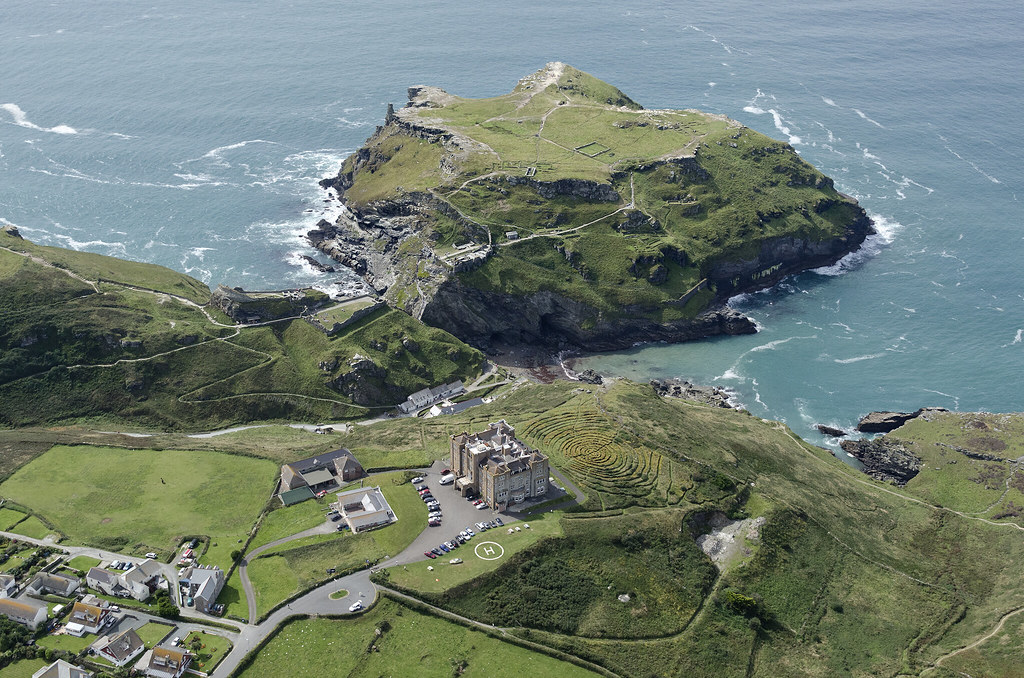This image is a high-angle aerial shot, likely taken by a drone or helicopter, showcasing a lush coastal landscape that appears to be in Scotland or Ireland. The scene centers around a large rock structure, covered in green grass, that juts out into the ocean and is connected to the mainland. Surrounding the rock, you can see ruins of old foundations, ancient farm walls, and remnants of old roads, indicating that it was possibly an outpost or grazing area in the past. Below the rock on the mainland, a well-maintained stone castle stands, and nearby is a prominent ancient concentric ring sculpture formed from stones. Adjacent to the castle is a helicopter pad marked with an "H," and further down into the valley by the ocean, there are several large white homes, possibly functioning as historical residences or hotels, with numerous cars parked around, indicating it is a popular location. The scene is very green with hills, valleys, and a backdrop of crashing ocean waves, evoking a distinctly Celtic vibe. The overall landscape is dotted with some residential buildings and shows a contrast between natural wilderness and human-made structures, all under a sunny sky with visible shadows and light reflections.